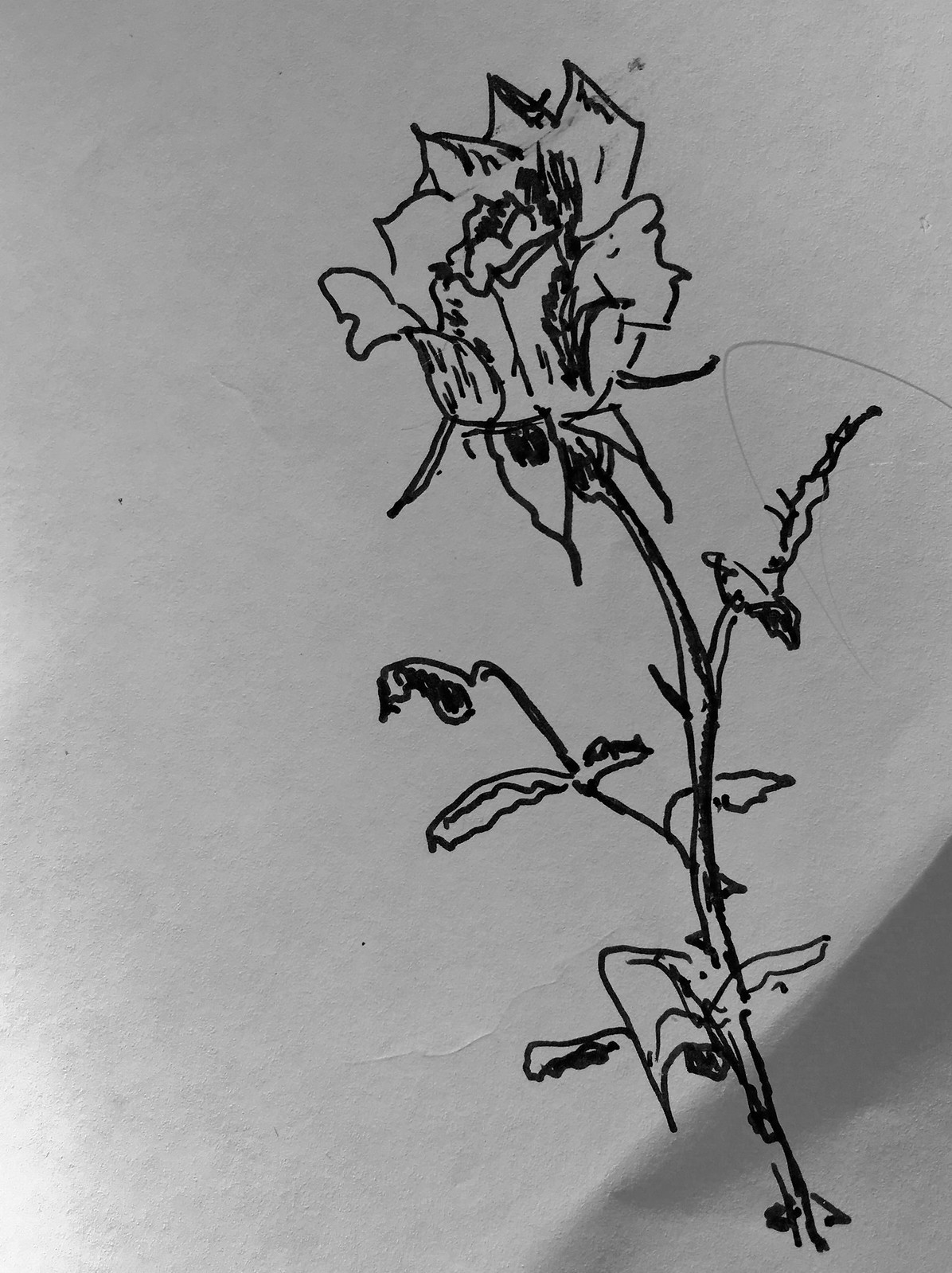This image depicts a detailed black-ink drawing of a rose on a slightly crinkled white piece of paper. The rose, leaning slightly towards the top left, is situated near the far right edge of the paper. The drawing, made with a black pen or marker, showcases pointed petals and a distinct center bloom, surrounded by additional downward-facing petals. The long stem extends from the bloom, featuring jagged leaves and thorns, complemented by extra pen marks to accentuate the intricate details of the petals and leaves. The photograph likely taken with a personal or cell phone camera, appears to be taller than it is wide, and shows some reflection in the bottom left corner, adding a sense of depth and realism to the representation.